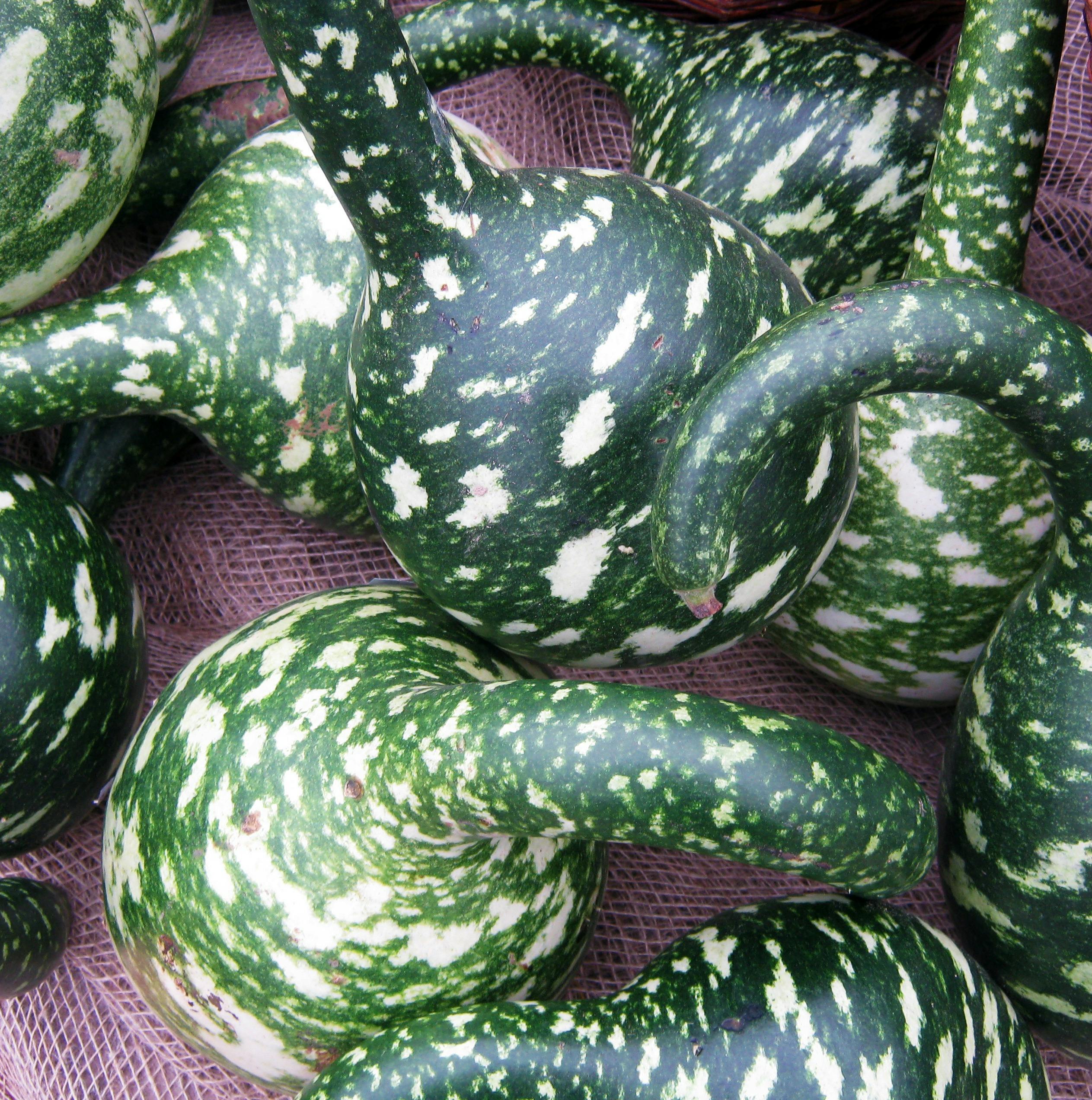The image showcases a close-up view of approximately ten green gourds, characterized by their spherical bases and elongated, curved necks resembling handles or horns. The gourds display a swirling pattern of dark and light green hues interspersed with white splotches that span their entire surface, including the distinctive necks. They are arranged on a canvas material that appears to be a tablecloth or netting in shades of lavender, violet, or pink. These healthy-looking gourds, likely squash, are perfectly ripe and possibly part of a display at a farmer's market, resting atop the colorful fabric backdrop.